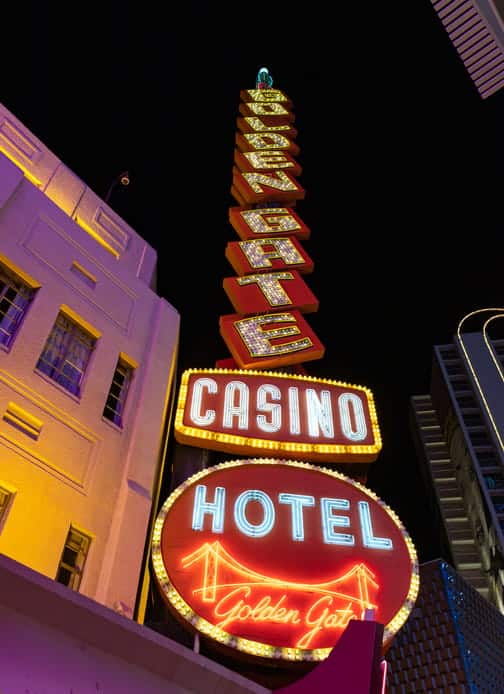In this nighttime photograph, a vivid neon sign for the Golden Gate Casino Hotel dominates the scene. The sign begins with vertical text spelling "Golden Gate," each letter individually framed and adorned with sparkling, glittery details that catch the eye, reminiscent of a disco ball. Below this, a horizontally oriented, rectangular light display reads "Casino" in striking white lettering against a red background, highlighted by golden lights. Beneath the casino sign, a circular light display features the word "Hotel" in bold white neon, surrounded by a radiant red circle with yellow lights bordering it. Below the hotel text, a depiction of the iconic Golden Gate Bridge is centered, with the name "Golden Gate" displayed in cursive beneath the bridge image. The scene is further accentuated by the stark contrast of the brightly illuminated signs against the dark night sky. Adjacent to the sign, part of a white hotel tower is visible, featuring several windows with faintly visible curtains. The view is angled from the perspective of someone standing on the ground, looking up at this vibrant display.